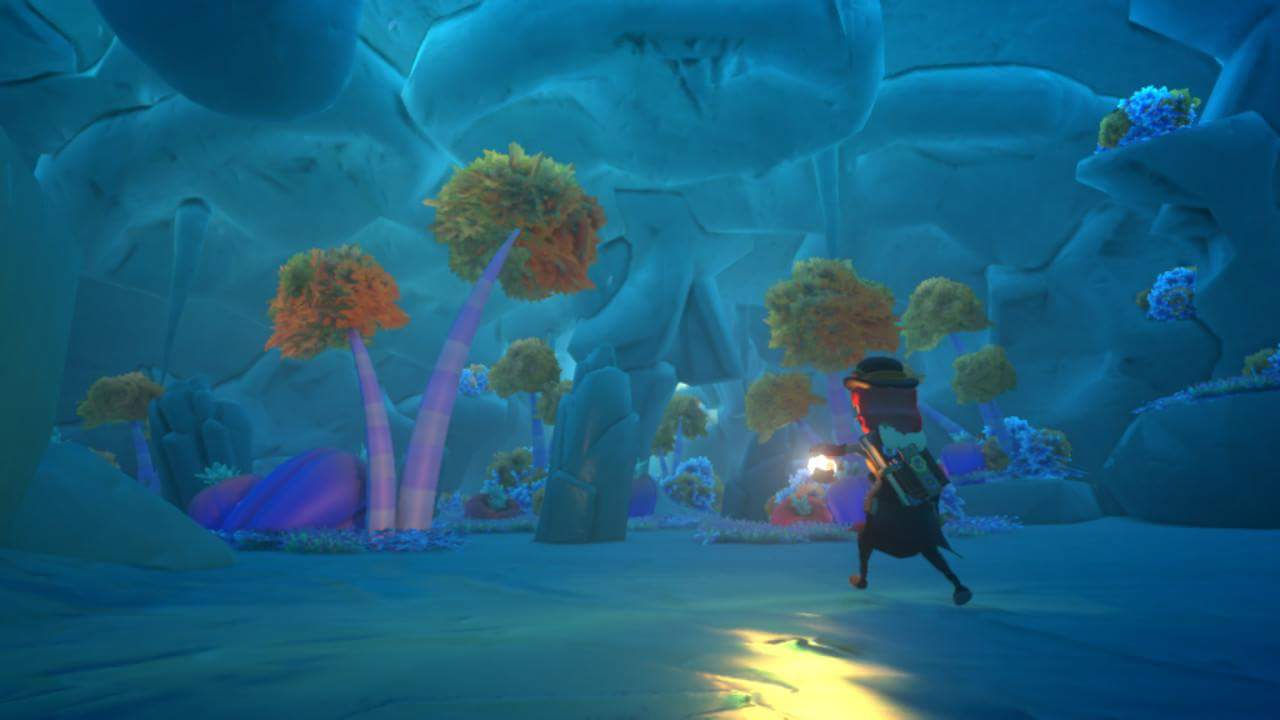The image showcases a screenshot from a video game set in a uniquely themed forest that combines elements of both ice and woodland environments. Dominated by cool blue tones, the scene evokes a cold, mystical atmosphere. At the center, dense trees and plants frame a small, shadowy entrance, towards which the character is walking. To illuminate the path, the character is holding a lantern, casting a faint glow on their immediate surroundings. The character is viewed from behind, wearing a distinctive hat and sporting long, pink hair, suggesting a female protagonist. The interplay of light and shadow, along with the blend of icy and forest elements, creates a visually intriguing and immersive scene.